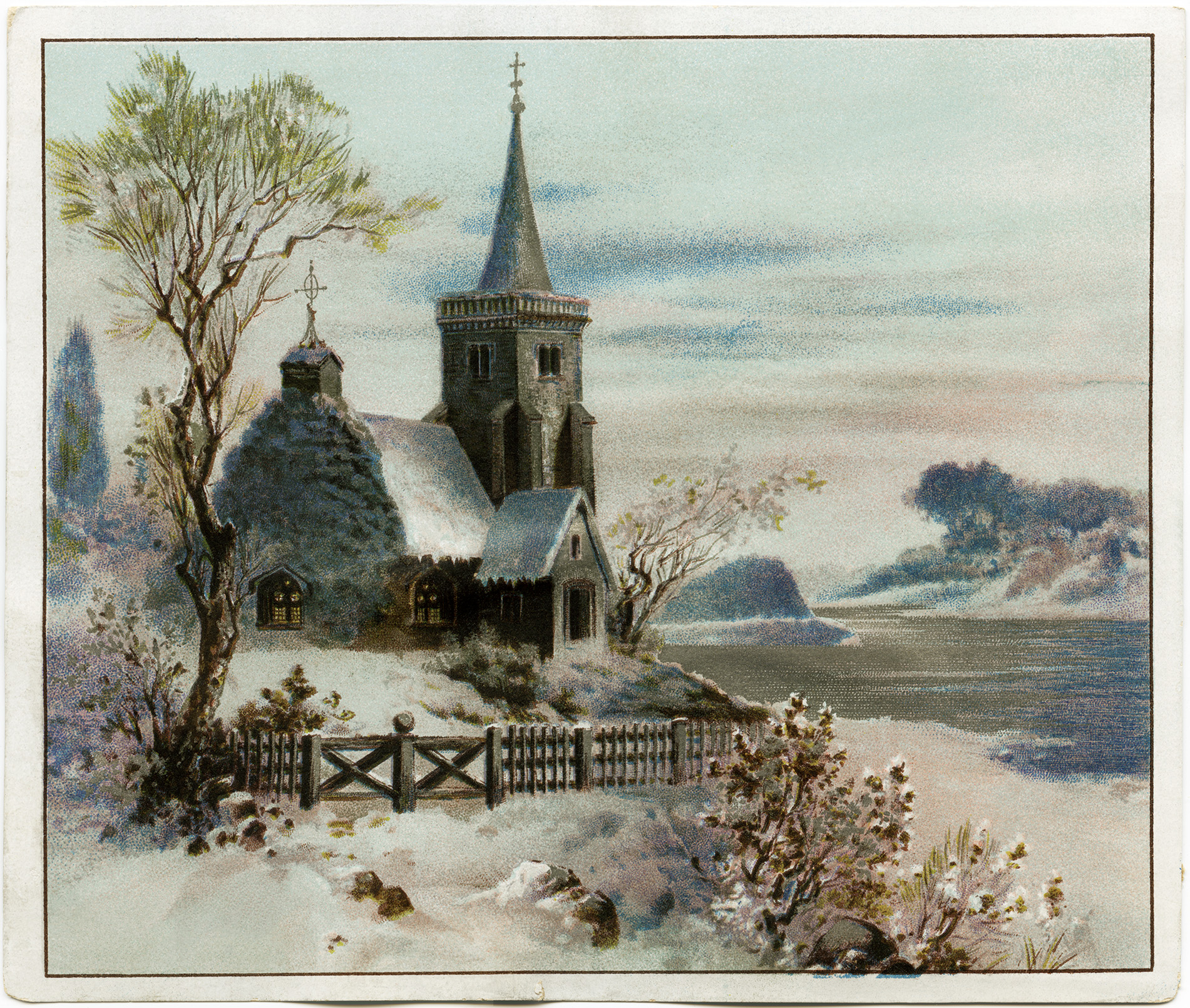This detailed painting portrays a serene, professional depiction of a quaint, old-fashioned chapel or church nestled in a winter landscape. The small, cottage-like structure is centrally positioned on a hill, slightly skewed to the left, with a tall, pointed steeple crowned by a cross, and an additional smaller steeple also adorned with a cross. A thick blanket of snow envelops the church's roof and surrounding ground, dominating the scene with white hues that contrast against the grey sky and muted tones of blue, grey, and brown seen throughout the image.

To the right of the chapel lies a body of water, possibly a pond or river, contributing to the tranquil ambiance. Hills rise in the background, dotted with trees and plants that peek out from the snow. A greyish-brown wooden fence encircles the chapel, adding to its old-world charm.

Illuminating through the wintery gloom, the church's round windows emit a soft, yellow glow, hinting at a warm interior presence. The scene is further softened by various flora—a tall, fern-like tree stands to the left, its green leaves partially visible amidst the snowy landscape, while white-flowered bushes and other shrubs covered in snow populate the right side, enhancing the picturesque quality of this wintery, artistic image. There's no text or artist's name present on the painting, which elevates the focus solely on the soothing, pretty depiction of this peaceful church scene.